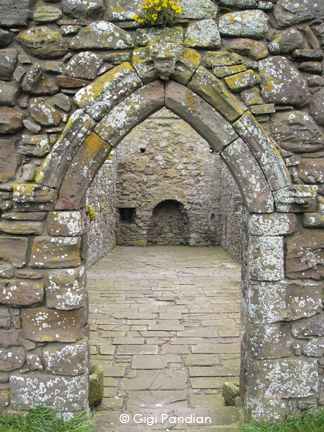The image captures the ancient ruins of a once grand and palatial structure, now a historical heritage site. The focal point is a striking, gothic-style arched entrance, constructed from rough, unevenly sized stones meticulously fitted together. The facade shows signs of age and weathering, adorned with patches of efflorescence, moss, and even some flora, including flowers emerging from the cracks in the stone. Beyond the arched gateway, a small stone room is visible, its floor paved with irregular stone slabs, and its walls featuring another rounded arch recess. The ambiance is further enriched by the scattered white and yellow spots on the weathered stone walls and the lush greenery, with plants and grass thriving at the base. A watermark at the bottom center reads "copyright Gigi Pandian," ensuring the image's authenticity and artistic ownership.